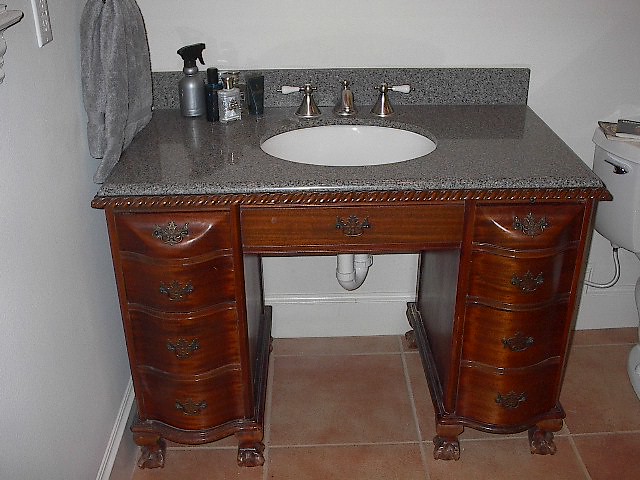The horizontal image showcases an antique-style vanity nestled in the corner of a bathroom. The vanity is adorned with a porcelain sink bowl and features a stainless steel faucet with a polished satin finish. The hot and cold water taps each have elegant white ceramic handles. The countertop is a gray granite finish, which seamlessly continues into a matching backsplash.

On the countertop, there are a few items: a semi-opaque glass bottle with a silver-colored cap and a white label, and a short stainless steel spray bottle with a black spray nozzle. A gray towel can be seen hanging on the white wall to the left of the vanity.

The vanity, crafted from antique mahogany wood, boasts ornate antique brass drawer pulls. It is supported by eight claw-foot legs and includes a total of six drawers, three on each side. Part of a white toilet tank is visible to the right of the vanity, indicating the layout of the room. The vanity sits on a floor of large red square tiles, and the room is bordered by a white baseboard.